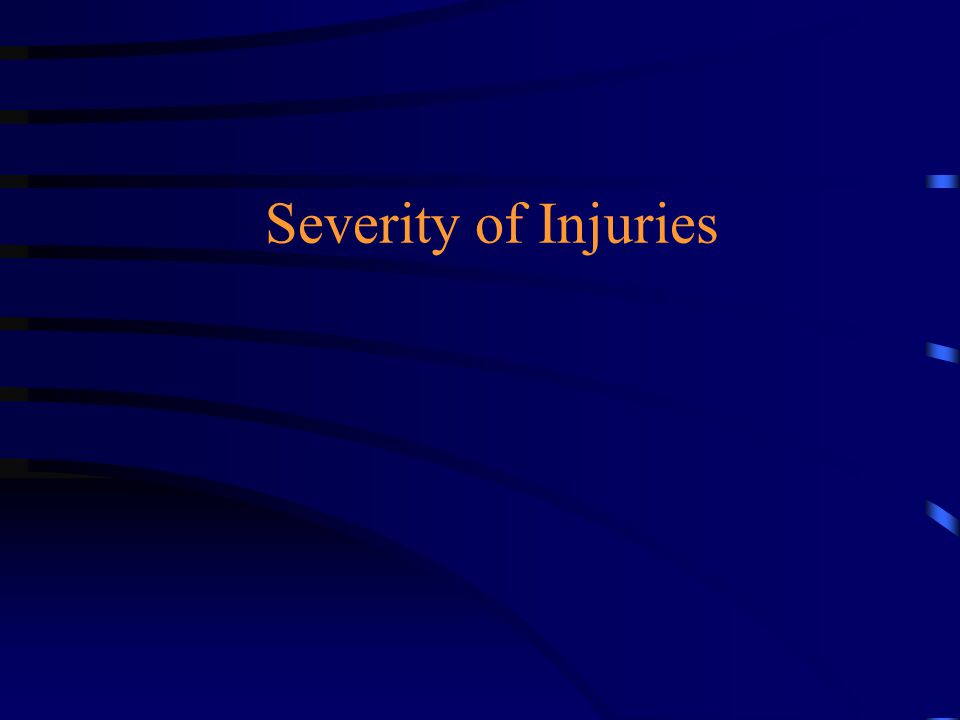The image resembles a PowerPoint presentation slide with a central, slightly elevated square area. The background is a dark blue or purplish-blue color, accented by horizontal black lines that curve slightly as they traverse the image. These lines vary in intensity and fade on the right side. Unique to the background are three small light blue dashes aligned vertically in the upper, central, and lower sections on the left side, mirrored by three lighter blue marks on the far right. Dominating the slide is a bold, centralized text in orange to yellow gradient letters reading, "Severity of Injuries." The text is positioned approximately in the upper two-thirds of the square area, standing out starkly against the dark, varied blue tones of the background. No additional text or graphic elements are present.